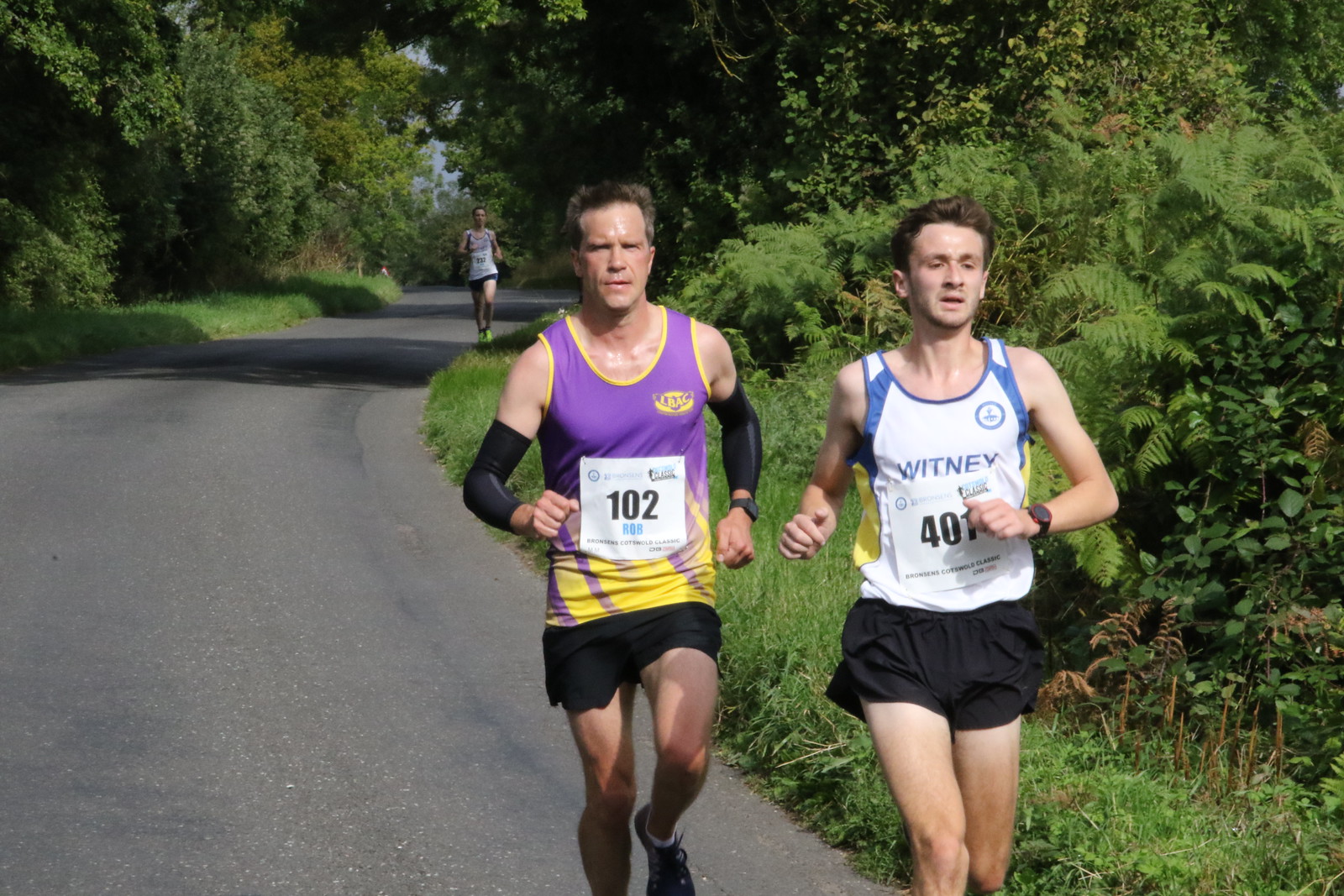This photograph captures a tranquil marathon scene set on a sunny day in the countryside. The path, a clean, paved road, winds through a lush, forested area surrounded by green grass, trees, and abundant vegetation on both sides. The image prominently features three runners. In the foreground, a man with dark hair, wearing a white tank top with blue and yellow trim, black shorts, and the number 401, leads the pack. Close behind, slightly to his left, is an older, square-jawed man in a purple tank top with yellow accents, black sleeves over his elbows, black shorts, and the number 102 displayed on his torso. In the distance, partially obscured by a bend in the road, a third runner, possibly female, can be seen chasing them, donning a white tank top, dark shorts, and bright green shoes. The scene exudes a serene and pleasant atmosphere under the clear, sunny sky.